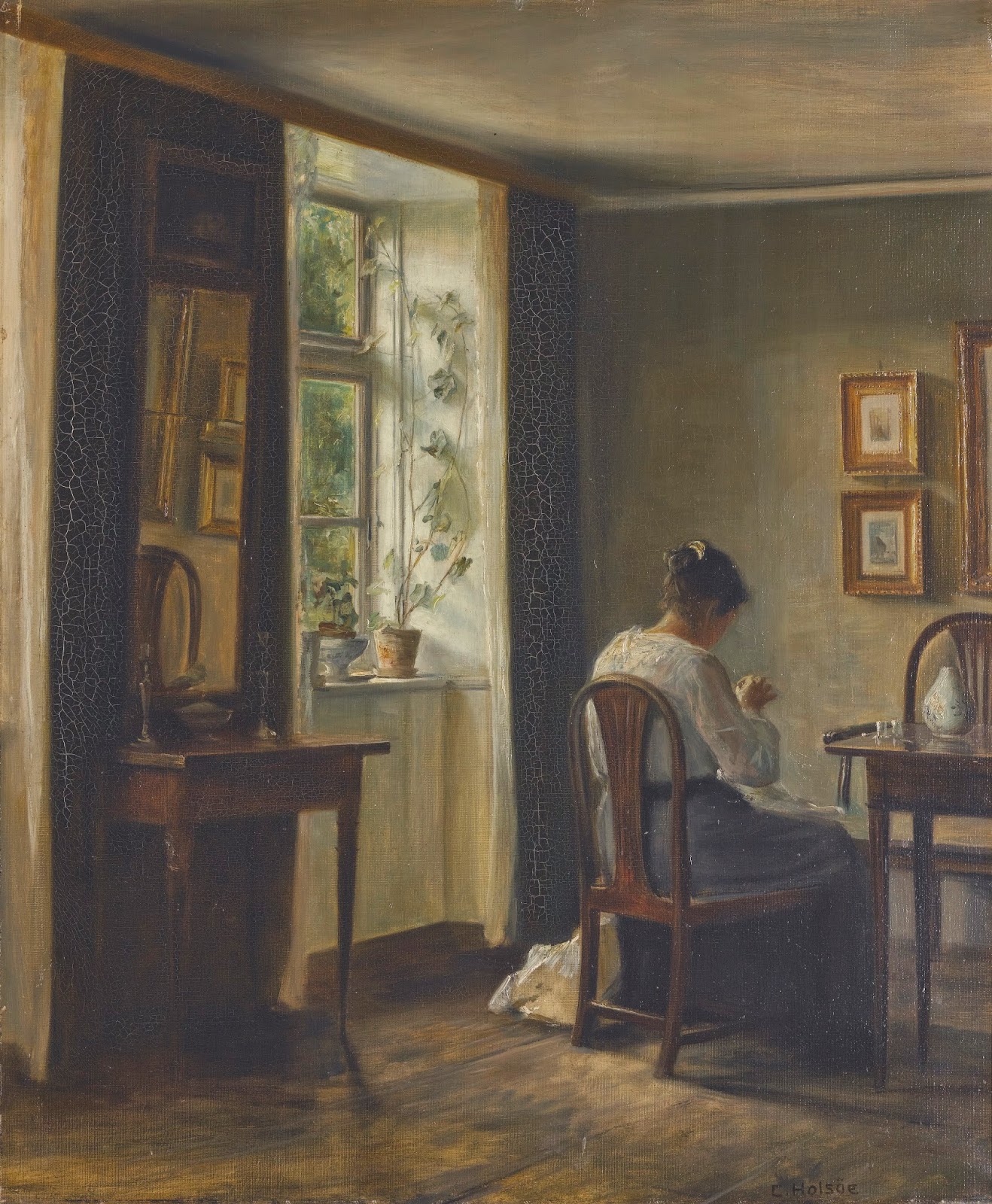The image is a detailed painting with warm colors, prominently featuring hues of green and brown, set in a vertical rectangular format. The main focus of the painting is a woman situated on the right-hand side. She is seated on an old wooden chair with her back to the viewer, facing slightly to the right. She appears to be engaged in intricate needlework, holding an item delicately between her index finger and thumb, while a piece of fabric extends from her lap all the way to the floor. Her posture is slightly slouched as she looks down at her hands, deeply absorbed in her activity.

In the background, directly in front of her, there's a brownish wall adorned with several framed pictures. To her right, a small wooden table holds an indiscernible object. To her left, there's a window with curtains, featuring tall potted plants resting on the windowsill. Adjacent to the window, there's a mirror on the wall with a small wooden stand placed in front of it. The entire room is accented by a hardwood floor, enhancing the painting's old-style ambiance.